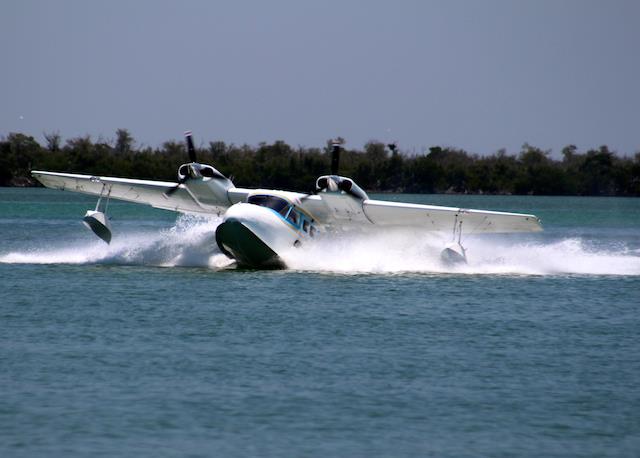The image depicts a small, white seaplane with blue accents around its windows, landing or taking off on a calm, blue body of water. The water, stretching from the bottom of the frame to about two-thirds up, ripples around the plane, creating white foam and splash. The plane's two propellers, mounted on top of the wings, appear in motion, suggested by a slight blur. The seaplane's nose points slightly upward, hinting at an ascent or gentle landing. The background showcases a dark, silhouetted treeline spanning from left to right under a medium blue sky. The scene is bright, with sunlight enhancing the clarity of the plane and water, while the overall simple nature of the image directs focus to the seaplane at the center.